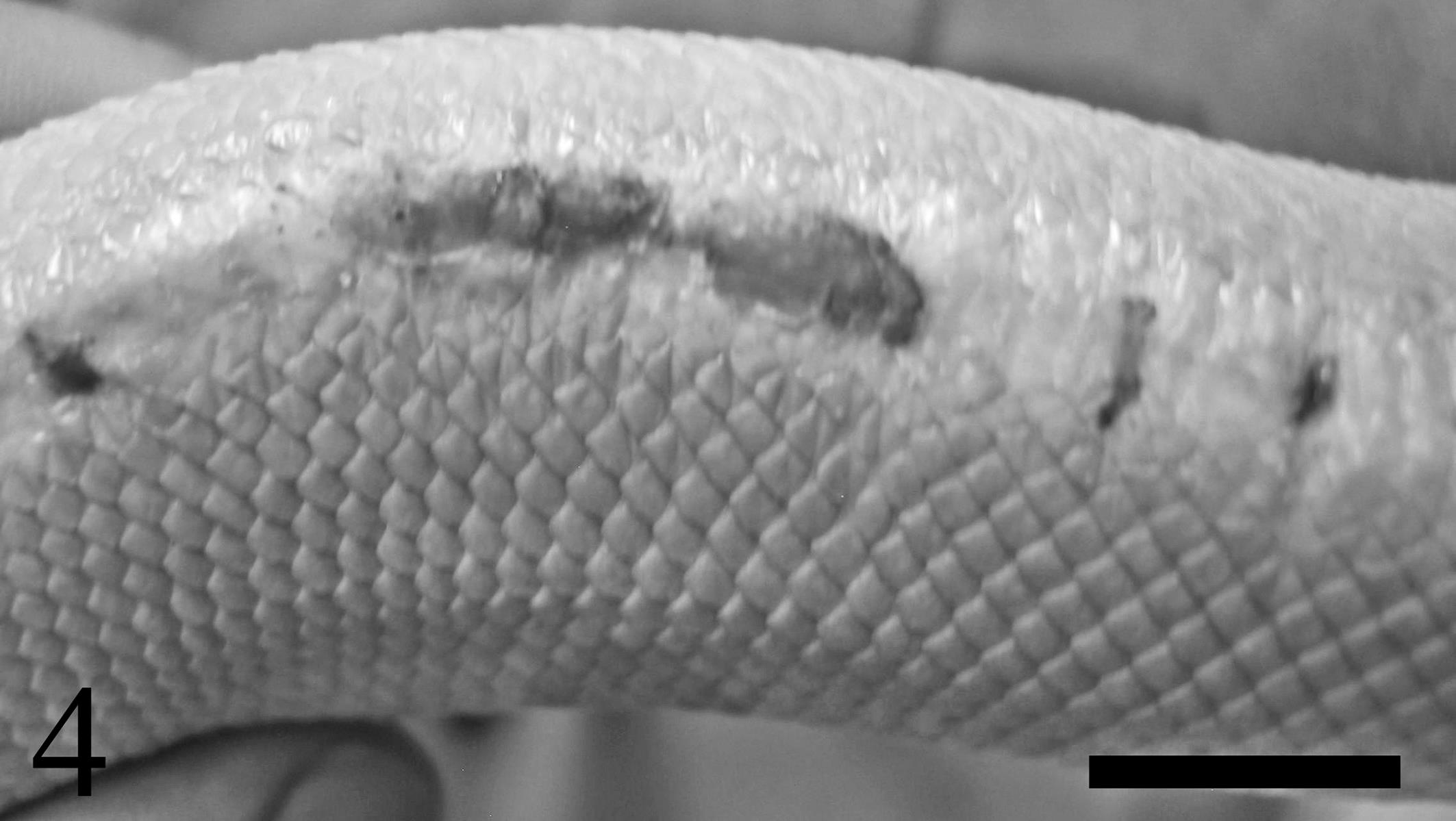This black-and-white photograph offers a detailed, up-close view of a thick, partially visible snake. The snake's body enters the frame at the top left corner, meandering downwards and slightly to the right until it exits halfway between the top and middle of the right edge of the image. The scales on the upper part of the snake appear smoother, interspersed with patches of dark spots, while the lower part reveals a more textured scaly surface. The overall coloration is light, possibly white or cream, with brown blotches visible along the body. In the bottom left corner, the photograph features a prominent black number four, with the tip of a person's finger or thumb, including the fingernail, subtly peeking from beneath the snake. The image concludes with a black rectangular bar positioned horizontally in the bottom right corner, cutting off the view of the snake's trailing body.